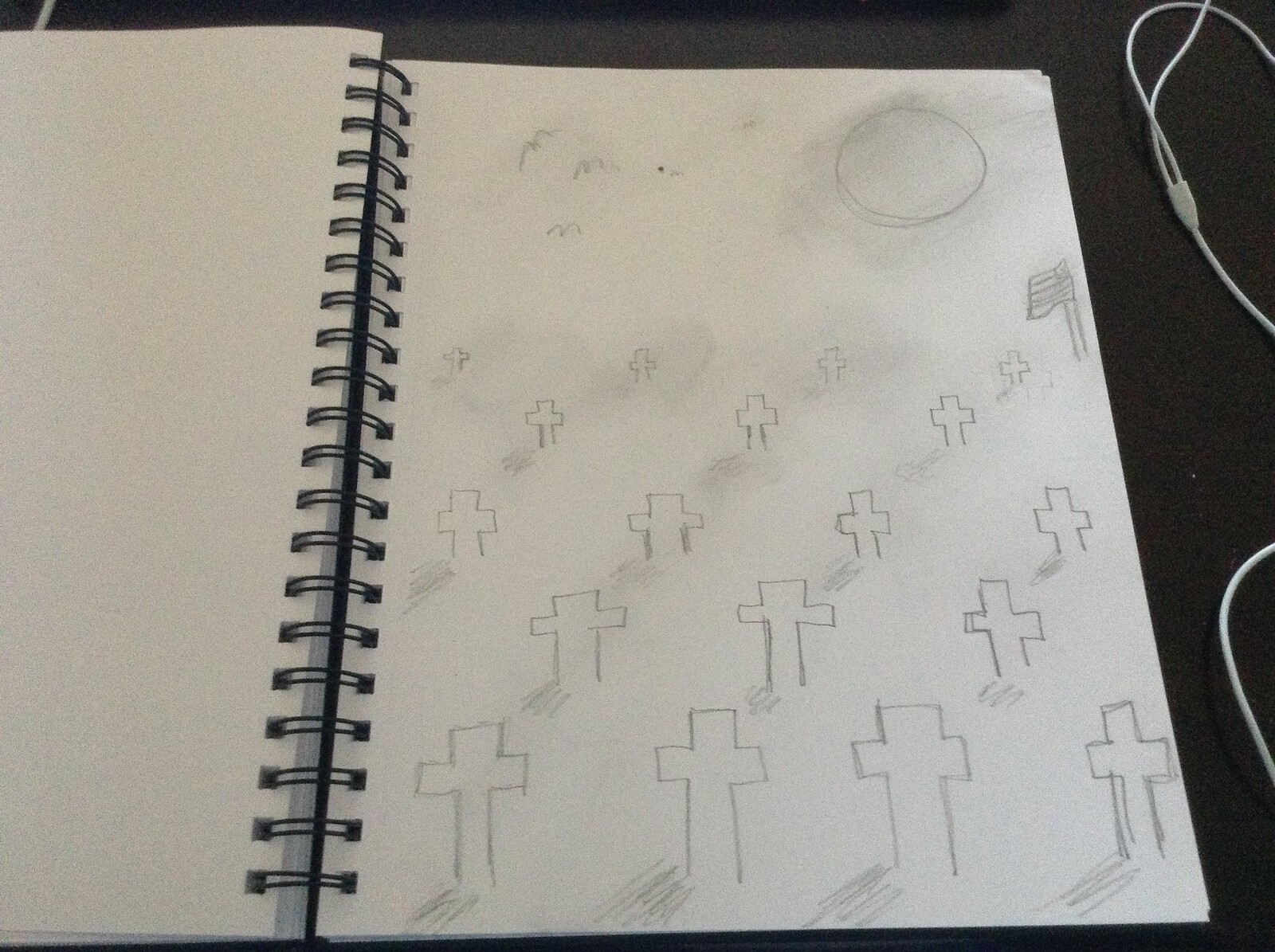The image features an open artist's sketchbook, spread across a black surface, likely a desk. The sketchbook, held together by black spiral bindings, shows a full page on the right and a partial page on the left, both of which are plain and unlined. On the right-hand page, there's a detailed pencil or charcoal drawing of a military cemetery, characterized by numerous rows of crosses that progressively diminish in size to indicate depth. Each cross casts a small shadow to its left. In the background, there is a large circular shape, potentially a sun or moon, without rays, and birds or bats flying in an 'M' formation. Additionally, an American flag appears to be waving in the wind on the right side of the drawing. Eraser marks and smudges suggest the artist's iterative process. On the right edge of the image, a white or light gray cord, perhaps from headphones, rests atop the sketchbook.